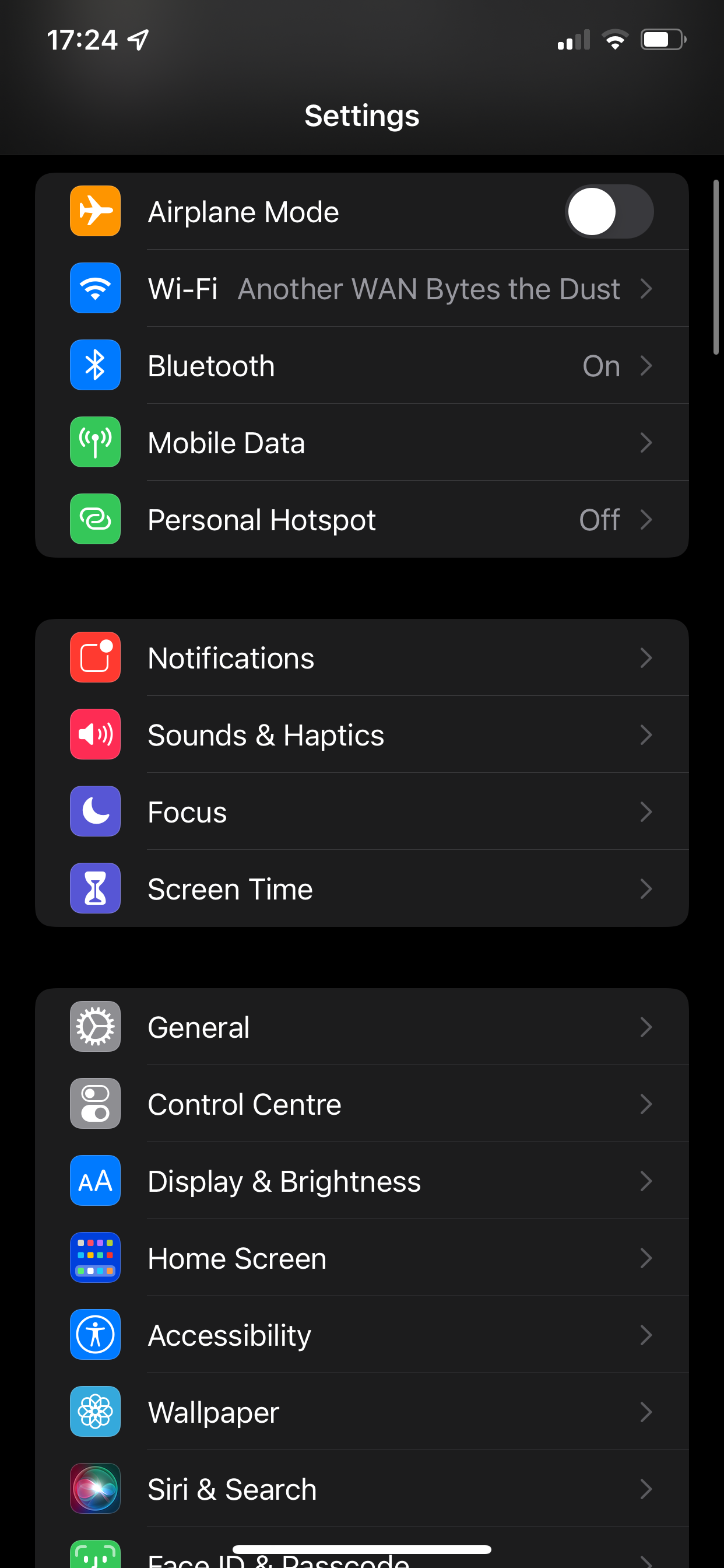This screenshot showcases the settings page on a smartphone. The display features a sleek black background with white font, ensuring high contrast and readability. At the top, the status bar indicates the current time as 17:24 on the left, while the right side displays a nearly full battery icon and signal bars in white.

The settings are organized into three distinct charcoal gray blocks, each containing multiple items accompanied by easily recognizable icons. 

In the first block:
1. Airplane Mode - Represented by an orange square with a white airplane icon.
2. Wi-Fi - Illustrated with curved lines on a blue background.
3. Bluetooth - Shown as a "B" icon on a blue background.
4. Mobile Data - Depicted by a tower emitting radio signals on a green background.
5. Personal Hotspot - Marked by a green square. 

Notably, all settings in this block are currently turned off.

The second block includes:
1. Notifications - Denoted by a square with a white dot in the top right corner.
2. Sounds & Haptics - Represented by a speaker emitting sound waves on a red background.
3. Focus - Illustrated with a crescent moon on a blue background.
4. Screen Time - Shown as a sand timer icon.

The third block encompasses:
1. General - Represented by a gear wheel icon on a gray background.
2. Control Center - Depicted with toggle switches, one on and one off, on a gray background.
3. Display & Brightness - Illustrated with two capital "A"s on a blue background.
4. Home Screen - Shown as colorful dots on a blue background.
5. Accessibility - Represented by a person within a circle on a turquoise background.
6. Wallpaper - Depicted by a flower on a turquoise background.
7. Siri & Search - Illustrated with the multicolored Siri waveform icon.

This detailed and organized layout provides easy navigation through the various settings on the device.